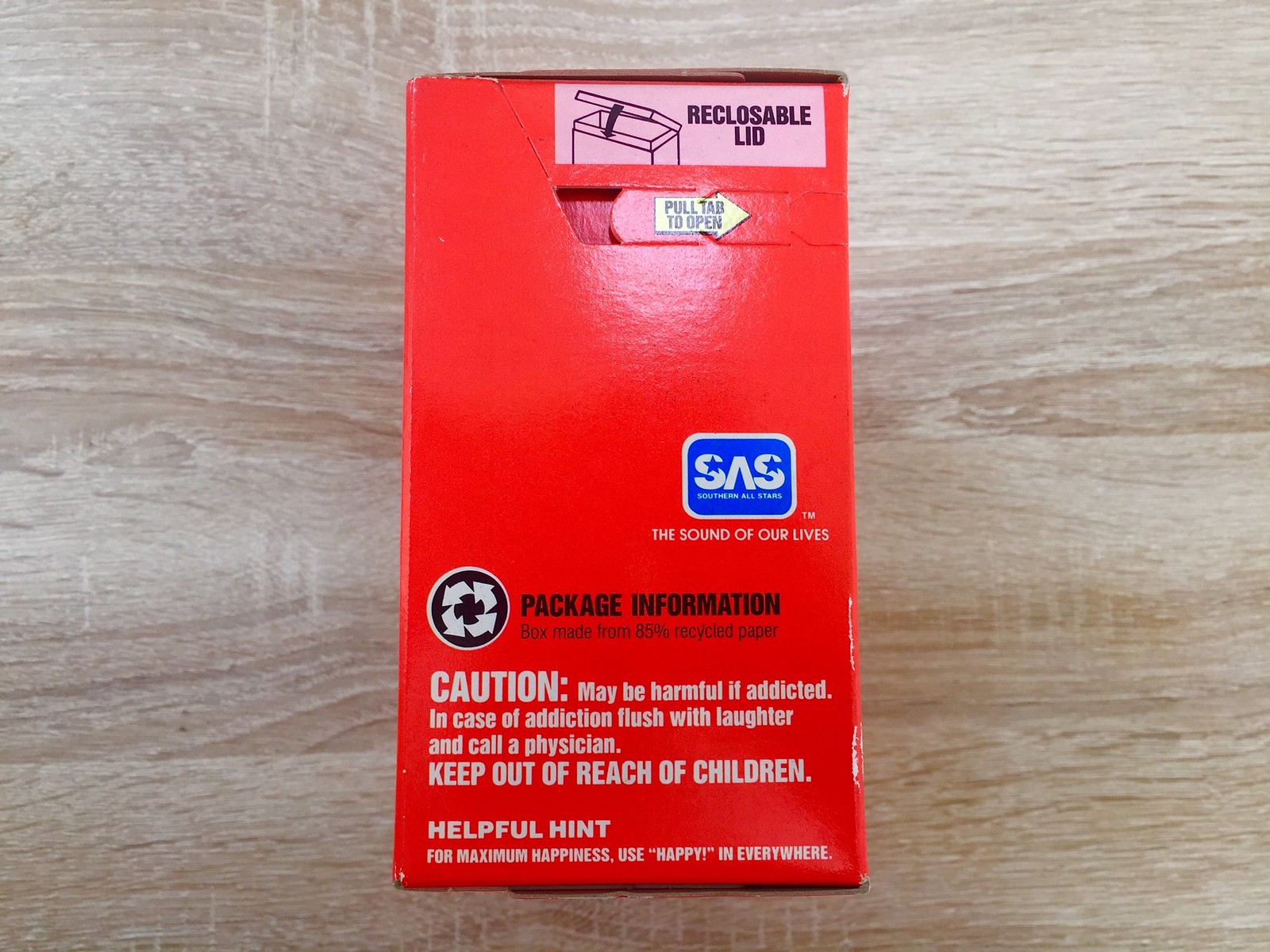The horizontally rectangular image features the back of a product box placed on a light tan wood grain background. The main color of the box is red. At the top right corner of the box, there's a pink banner with black text that reads "Reclosable Lid." Directly beneath this banner is a horizontal perforated section labeled "Pull Tab to Open."

Further down on the right side, a small blue square with a white border and white lettering displays the initials "SAS." Spanning the bottom portion of the box, from left to right, is a large block of text under the heading "Package Information." It states: 
"Box made from 85% recycled paper. Caution, may be harmful if addicted. In case of addiction, flush with laughter and call a physician. Keep out of reach of children. Helpful hint, for maximum happiness, use Happy in everywhere."